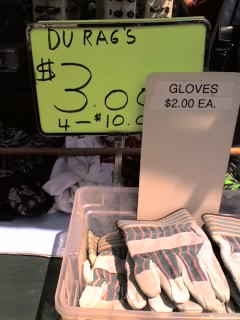The image depicts a scene likely taken at an outdoor market or shop. At the bottom, partially visible, is a clear pinkish Tupperware bin filled with tan, striped gardening gloves. A neatly printed label on tan cardboard in black letters reads, "Gloves, $2 each," attached to the bin. Behind this, a bright neon yellow handwritten sign is displayed within a metal frame, announcing "Do rags, $3" with an additional offer, "4 for $10," although part of this sign is obscured by the gloves sign. Sunlight casts shadows across the scene, indicating it is outdoors. In the background, a metal barrier partially conceals other folded materials, likely the do-rags mentioned in the sign.